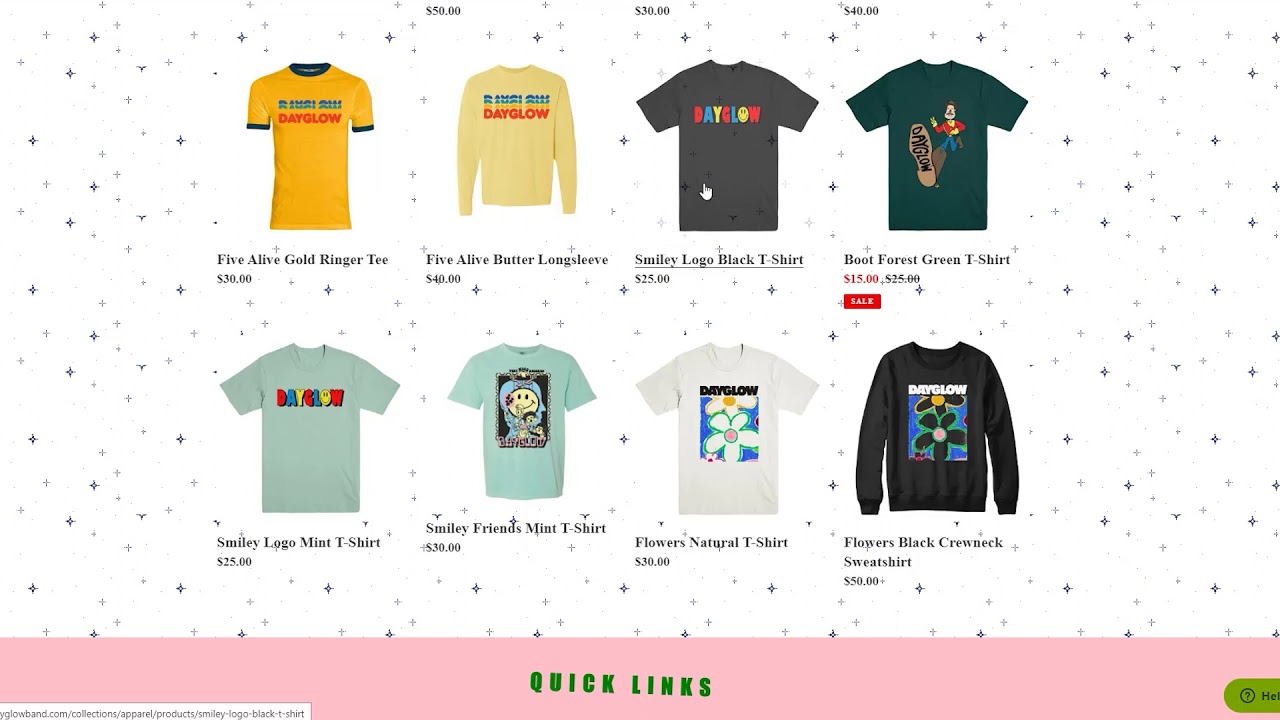This image captures a clothing website interface featuring a vibrant mix of graphic elements and product details. At the bottom, there is a slightly tilted, bold green banner labeled "Quick Links" on a pink rectangular background, suggesting a touch of whimsical design, though its alignment appears slightly off. To the right, a partial view of a 'Help' sign is visible, while the left edge reveals a fragment of the website's URL.

The top portion showcases a variety of shirts against a backdrop adorned with black and white stars. There are approximately eight shirts displayed, each in a different color. Primary highlights include two long sleeve shirts, one in black and the other in a bright yellow with "Day Glow" printed on them. The collection also features a gold "Day Glow" shirt, a brown shirt, a sky green shirt, and a white one, each adorned with unique front images. The array offers a colorful and diverse selection, appealing to various style preferences.